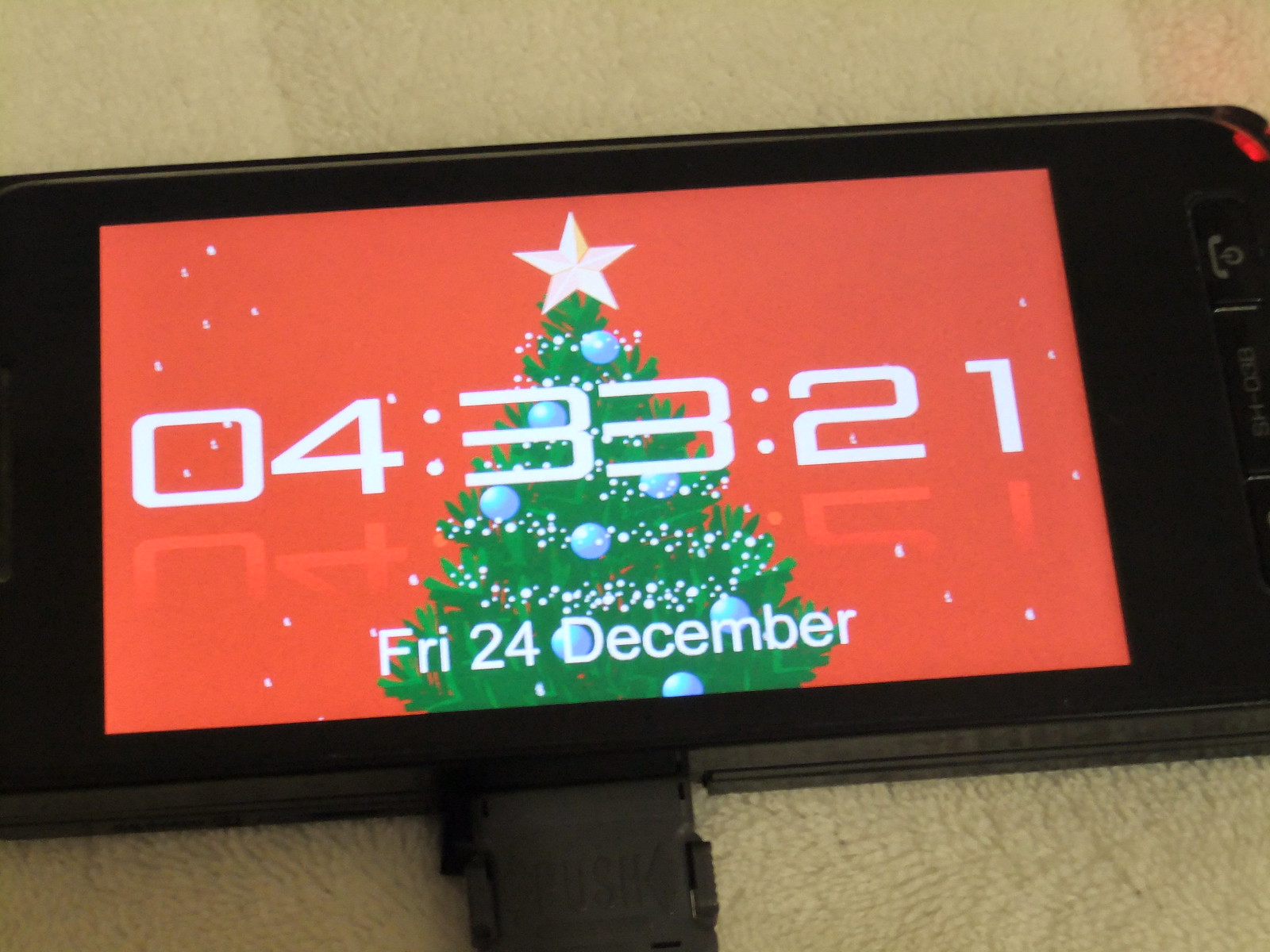This photograph features a black electronic device encased in a matching black cover, resting softly on a tan cushioned surface. The screen of the device displays a vibrant red-orange background adorned with white snowfall. Central to the screen is a festive green Christmas tree, decorated with white ball ornaments and twinkling white lights, topped with an elegant white star or eagle figure. Superimposed over the tree, in white font, is a sequence of numbers, "043321". Below this, the date "Friday, 24th of December" is also clearly displayed in white font, adding to the holiday theme of the image.